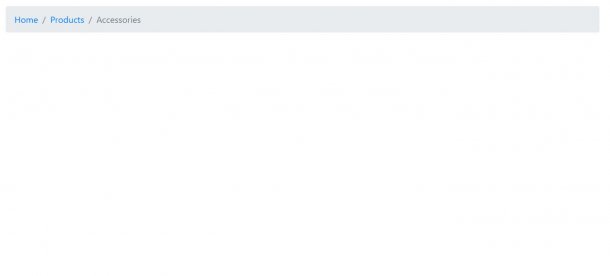This image predominantly features a plain white background, creating a minimalist appearance. Toward the top of the image, there is a thin, horizontal bar that stretches from the left edge to the right edge. This bar, colored in a medium to light gray, contains three clickable text options formatted with capitalized initial letters followed by lowercase letters.

On the far left of the bar, the word "Home" is presented in small, blue text, indicating it may be an active or previously clicked link. A gray slash separator follows, leading to the next option, "Products," also in small, blue text, suggesting it is another clickable link. Another gray slash separates "Products" from the final option, "Accessories," which appears in darker gray text, possibly indicating it is the current or an inactive link.

This structured header bar adds a subtle, yet clear navigation element to the otherwise entirely white and unadorned image.